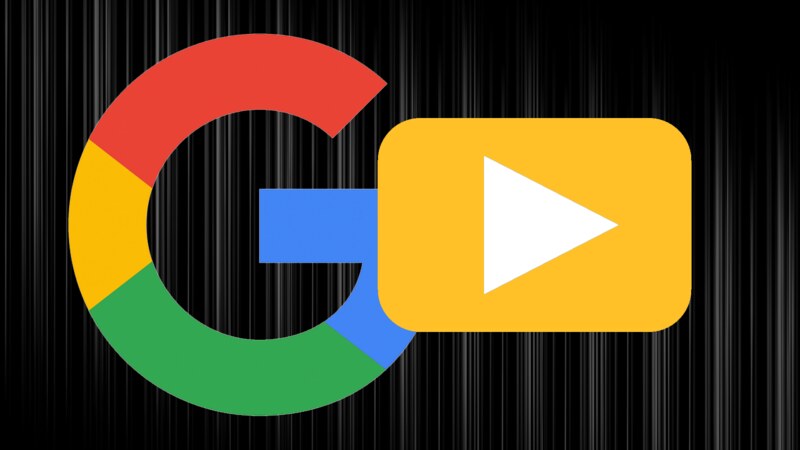This image features the iconic "G" logo representing Google, prominently displayed in large, vibrant colors: red, yellow, green, and blue. The "G" is detailed with precise color segmentation that seamlessly merges these hues. Positioned within the image is a prominent yellow circular button containing a sideways triangle, suggestive of a play button often associated with multimedia applications.

The entire scene is set against a striking black background embellished with vertical stripes of white and light gray, giving an impression reminiscent of elegant theater curtains. This background adds depth and sophistication, contrasting sharply with the dynamic colors of the Google logo and the playful yellow button.

Notably, there are no textual elements in the image, nor are there any additional graphic components, focusing the viewer's attention solely on the Google branding elements. The design suggests an app icon or a clickable interface element, highlighting how users could interact with it. The yellow behind the triangle slightly overlaps part of the blue in the "G," adding a subtle layer of visual interest and complexity to the composition.